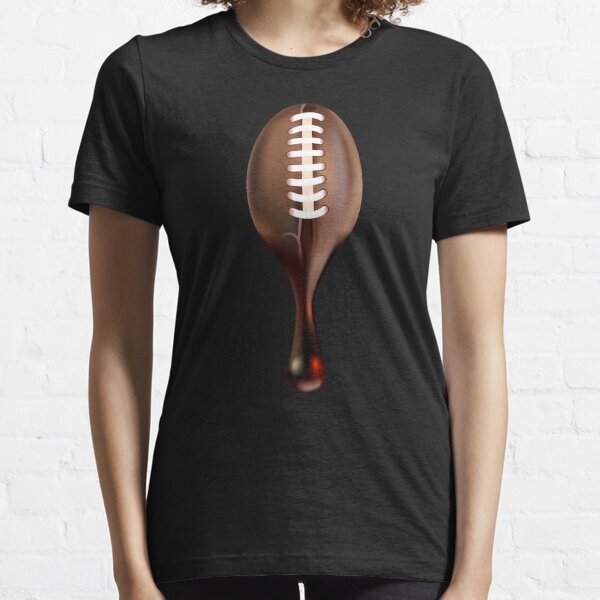This photograph features a woman with curly dark hair, whose face is cropped out, showcasing her from the neck down to her upper thighs. She is wearing a black cotton t-shirt that fits her loosely, with dark pants. The t-shirt has a unique design centered on the chest – a coffee bean made to resemble a football, complete with white stitching. This football-like coffee bean appears to bleed into a liquid drip, transitioning from a brown color to a reflective blood-red hue at the tip. The backdrop of the image is a white brick wall, adding a stark contrast to her dark attire. The woman appears to be either white or Latina.